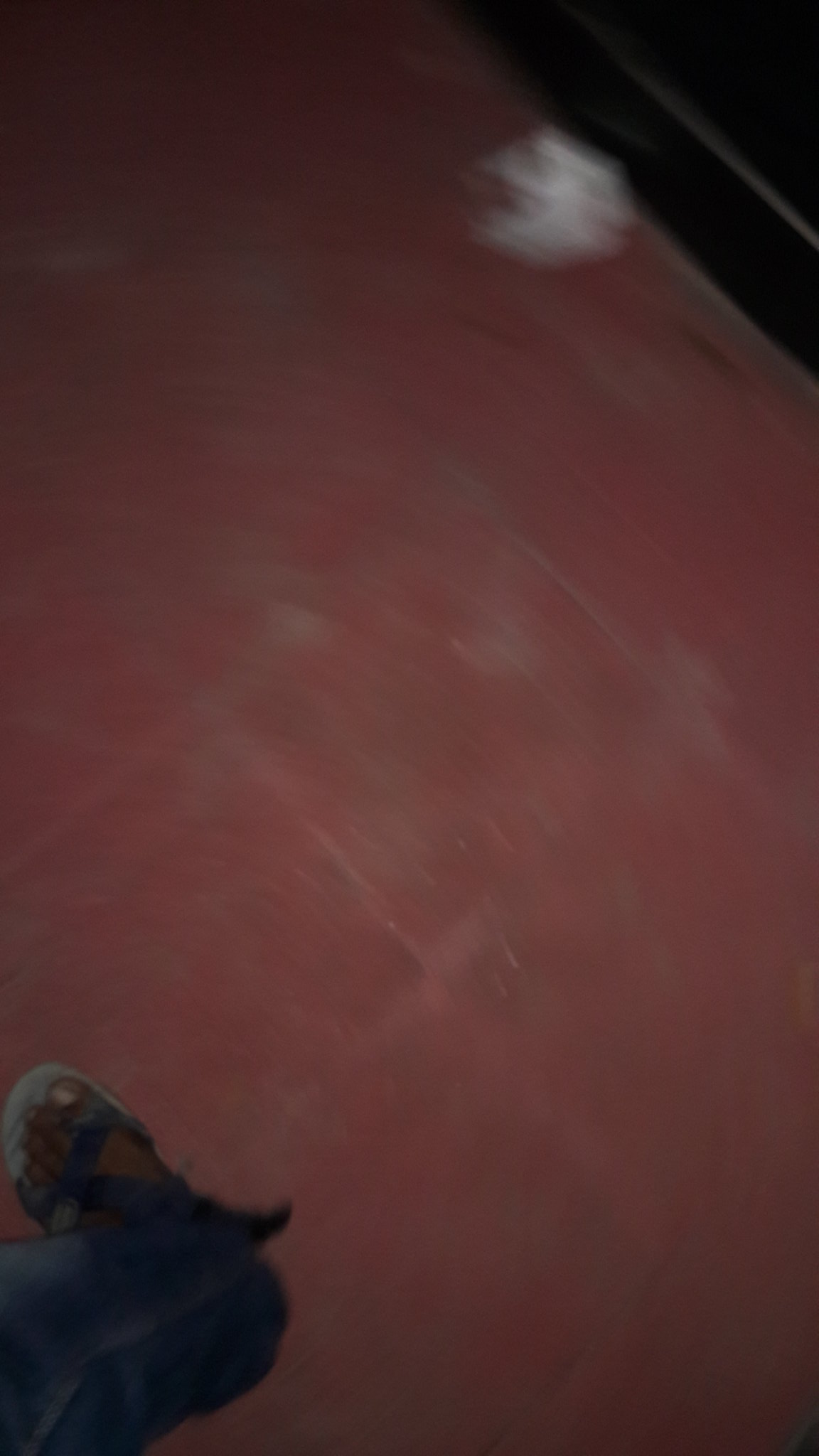The photo is a blurry, top-down shot of a red-tiled floor, with square tiles that resemble Mexican tiles. On the lower left-hand corner, there's a partial view of a person's right leg and foot, with the person wearing dark pants and a dark cross-strapped sandal. The tip of the sandal appears lighter, possibly due to dust or dirt. The floor tiles stretch across the image, revealing a worn and slightly rusted appearance in places. The grout lines between the tiles are not prominently visible.

At the top of the image, a black baseboard or possibly an edge of a counter runs diagonally, forming a triangular black shape in the upper right corner. Adjacent to this is a white, cloudy shape that might be debris or trash. The upper portion of the image includes a darker section suggestive of either a wall or counter edge, further enhancing the bustling and somewhat aged look of the setting.